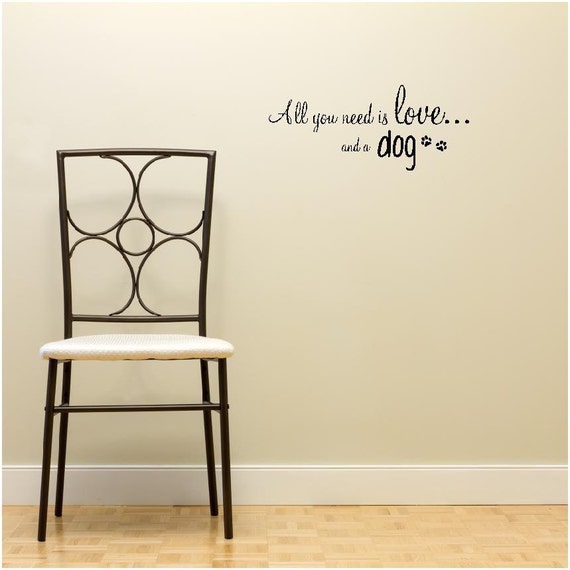This image portrays a minimalist setting featuring a chair positioned on the left side against a light tan wall adorned with the phrase "All you need is love... and a dog" in a black cursive font, with two black paw prints accompanying the word "dog." The chair has a simple design with a white cushion seat and an interesting geometric black metal frame, including a central circle and circles at each of the four corners of the backrest. The floor is a bright, reflective, light wood or faux hardwood, complemented by a tall white baseboard with subtle crown molding. The overall composition conveys a clean, modern, and serene atmosphere.